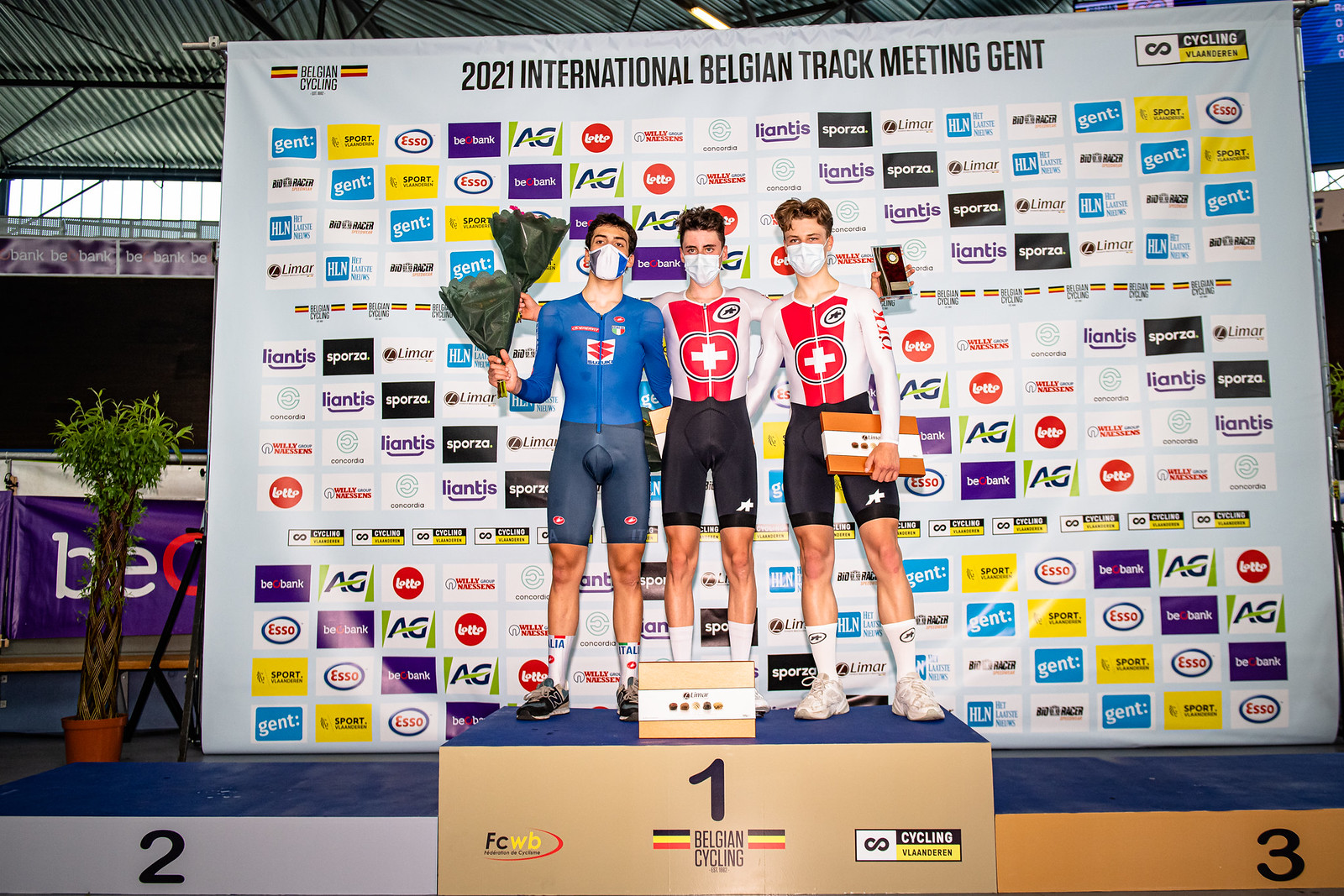The image captures the podium ceremony at the 2021 International Belgian Track Meeting in Gent. Three male athletes are standing on the podium, each in a designated spot, all wearing face masks. The athlete on the left is dressed in a blue cycling top with dark blue shorts, while the middle and right athletes are in identical white cycling tops featuring a red cross and the Swiss flag, paired with black shorts. All three are holding boxes of chocolates and the two athletes on the left are also holding bouquets of flowers. They are all dressed in cycling gear inclusive of high white socks and running shoes.

The backdrop is adorned with various sponsor logos such as Pazoria, Elancis, Iso, Gent, and HLM, arranged in small repeating rectangles. The large poster behind them prominently reads "2021 International Belgian Track Meeting Gent," establishing the event's location and nature. This appears to be a cycling event given the attire of the athletes and the mention of Belgian cycling, highlighted by logos and text in the background.